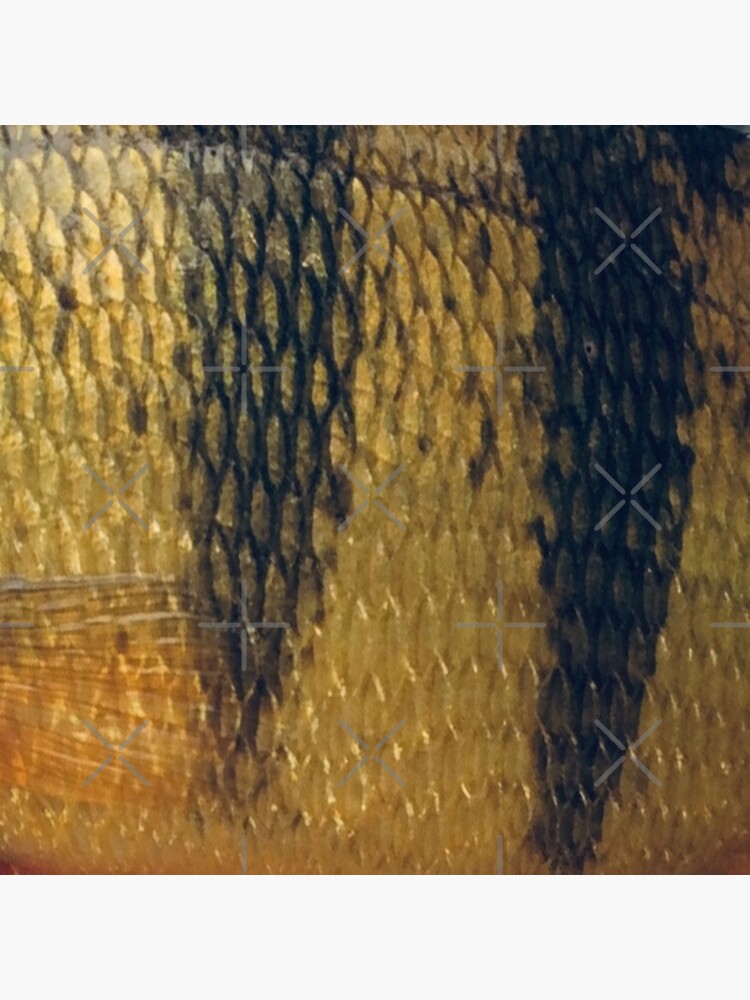This highly detailed close-up photograph showcases the intricate patterns and vibrant colors of what appears to be a fish, potentially a bumblebee cichlid or goldfish. Dominating the image are the fish's small, meticulously outlined scales, which exhibit a striking golden hue interspersed with darker, blackened scales. The scales are predominantly golden with some displaying a muddier yellow color. Particularly noticeable are the two prominent horizontal black stripes that cut across the fish's body. Adding to the complexity are three cross-hatched X marks over these black stripes, rendered in a light, semi-transparent color. The bottom left corner of the image reveals a portion of the fish's fin, detailed enough to show individual scales, highlighting its role in propelling the fish. The overall composition, with its mix of golden, yellow, and black hues, creates an almost prism-like effect, giving a sense of depth and transparency despite the close-up perspective. This fascinating visual is further complicated with subtle X and plus marks that overlay the pattern, as if the image were being examined through a camera lens or mapping grid.